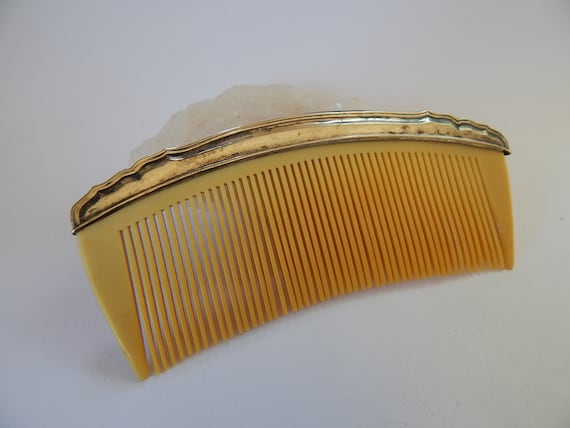This image showcases an antique hair comb likely from the 1920s, resting on a plain white background. The main body of the comb is a rich yellow with a slight orange tint, adorned with closely spaced, fine teeth, indicative of its purpose as a barrette or decorative hair accessory. Atop the comb, there's an ornately curved metallic piece, resembling aged silver or bronze, with distinct age markings that evoke a sense of vintage charm. Crowning this metal strip, there's a delicate, undefined ivory or white decoration, possibly a crystal, enhancing its antique aesthetic. The accessory's design suggests that when worn, the decorative metallic and ivory elements would be prominently visible, offering an elegant accent to a woman's hairstyle of that era.